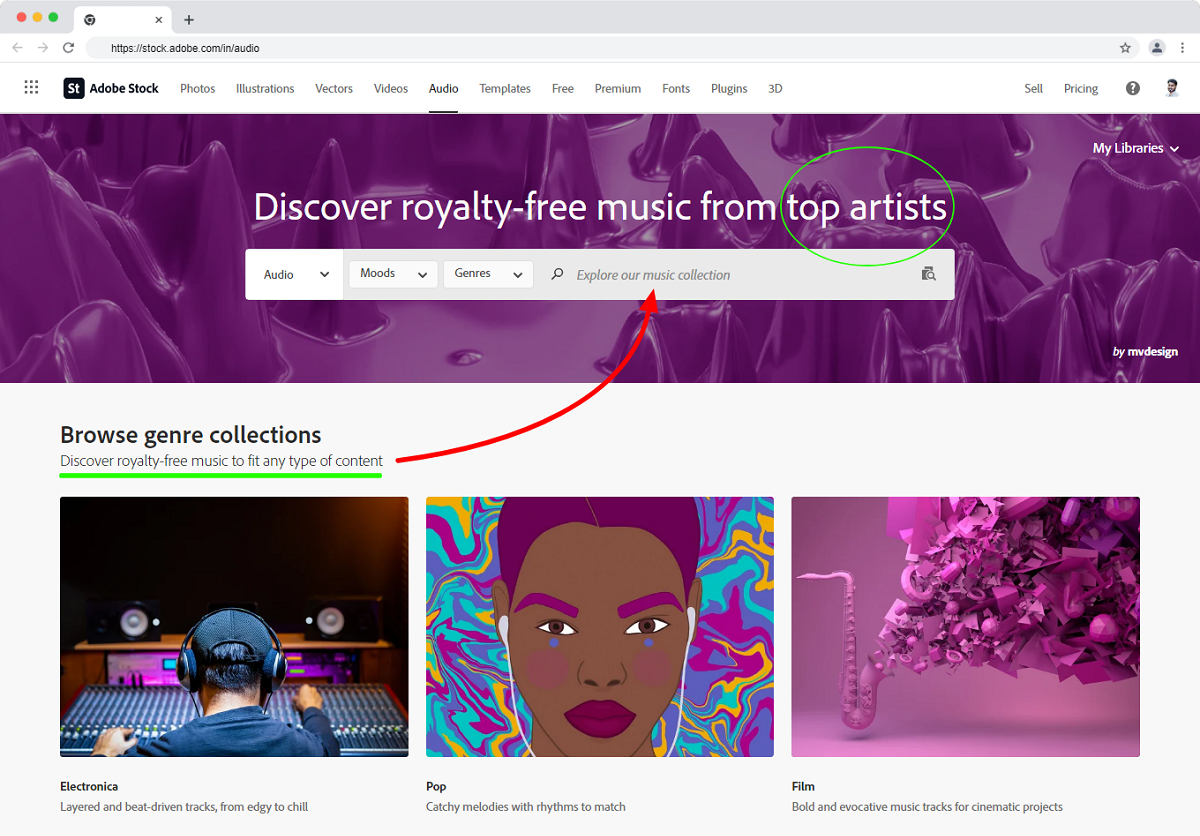The image showcases the music section of the Adobe Stock website, characterized by a minimalist color scheme of grey, white, and black, with some accent colors. The top bar includes various categories such as Photos, Illustrations, Vectors, Videos, Audio (which is currently selected), Templates, Free, Premium, Fonts, Plugins, and 3D. Additional buttons for Sell, Pricing, a question mark icon for help, and a small avatar of the signed-in user are also visible.

The header at the top of the page is in monochrome purple, reading "Discover royalty-free music from top artists," with "top artists" encircled in green. Beneath this is a search bar labeled with Audio, Moods, Genre, and a placeholder text saying "Explore our music collection."

The main section of the page features thumbnails categorized by genre: Electronics, Pop, and Film. Each thumbnail is annotated with descriptions: Electronics - "Layered and beat-driven tracks from edgy to chill"; Pop - "Catchy melodies with rhythm"; Film - "Bold and innovative, evocative music tracks for cinematic projects." The annotations also include added underlines in green and an upward-pointing red arrow for emphasis.

Overall, the page highlights Adobe Stock's royalty-free music collection, offering various genres to suit different content needs.